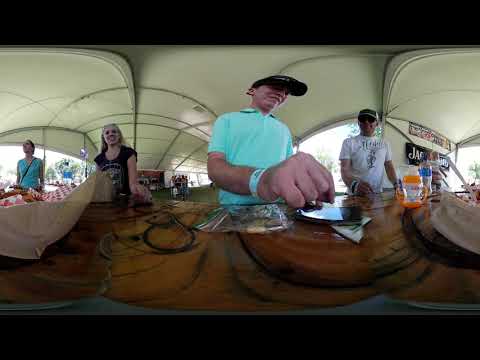In this panoramic 360-degree image, a group of people is gathered around a wooden countertop. The photo's wide-angle lens causes some distortion, making objects and hands appear unusually large. In the foreground, a man in a light green collared shirt and a black hat is engaging with his cell phone, possibly pushing a button. To his right, a man in a white short-sleeve shirt with a hat and glasses stands by. On the left side of the image, a woman wearing a blue sleeveless shirt and another woman in a black sleeveless shirt, who appears to be smiling, are visible. Another woman in a teal top is standing further left. Atop the wooden counter are various items, including a basket with food, a bottle of water, and an orange beverage. The scene is well-lit, with natural light streaming in through large windows in the background. There is also a tablecloth with a gingham-like design on one side of the countertop, adding a touch of homey decor to what appears to be a bustling yet cozy setting.